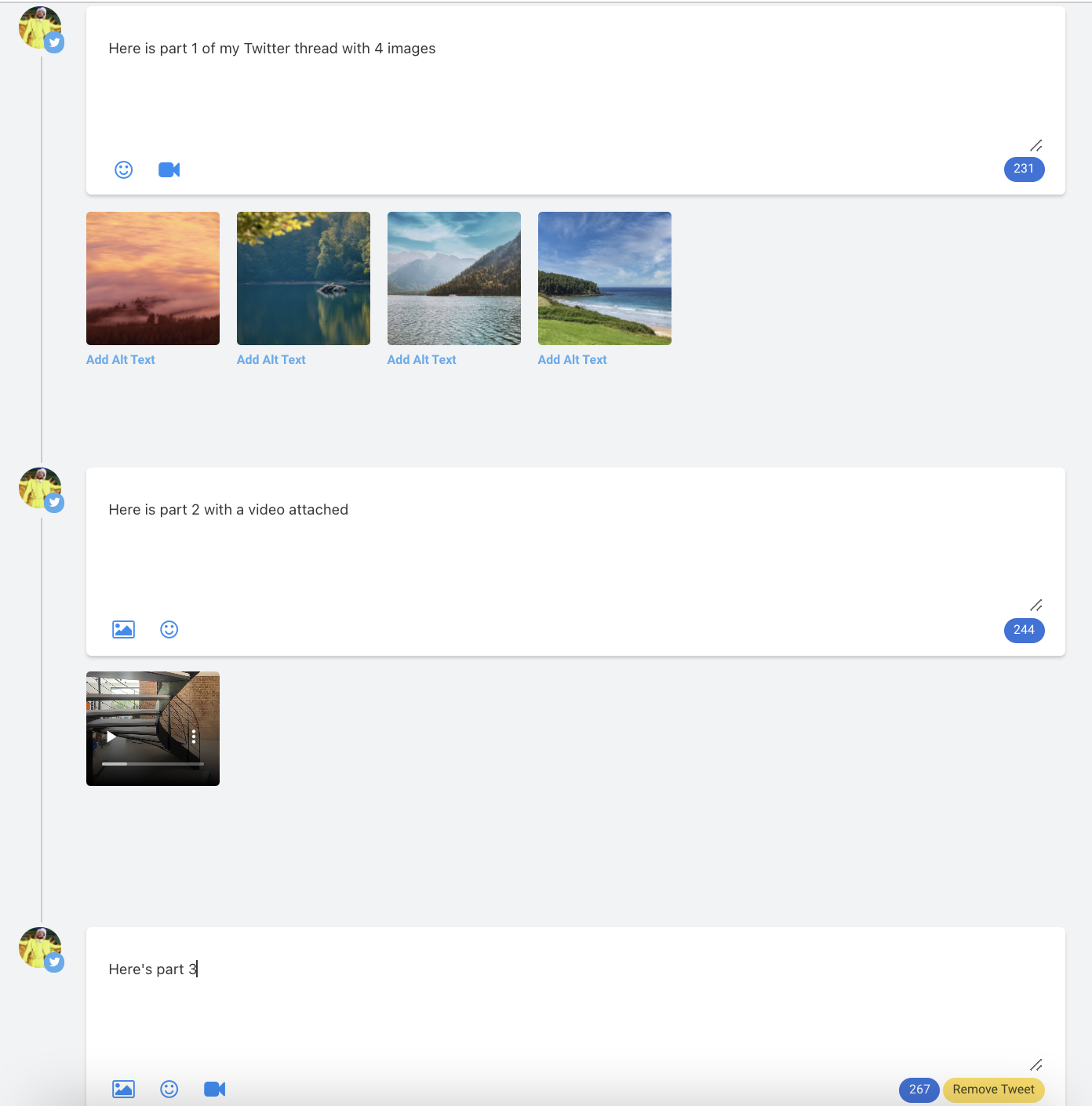The screenshot showcases a website resembling Twitter, featuring a social media network where users can share text, images, and videos. The image is set against a light gray background and contains three large, vertically stacked white boxes.

The top white box features black centered text reading, "Here is part one of my Twitter thread with four images." In the top left corner of this box, there is a profile picture—a small circle depicting a man wearing a yellow shirt. Adjacent to this profile picture, on its bottom right, is a blue circle with a bird emblem reminiscent of the Twitter logo. Below this box are four images with varied visuals: one displays striking red and orange clouds, while the other three capture serene outdoor scenes of lakes, mountains, grass, and clouds. Each of these four images includes blue text at the bottom prompting, "Add alt text."

The center white box mirrors the structure of the first but contains the text, "Here is part two," accompanied by a video. This video is represented by a thumbnail image featuring a white play button in the center and a seek bar at the bottom.

The bottom white box starts with the text, "Here is part three." However, the lower portion of this box is cut off, leaving the remainder hidden from view. This signifies that it is the third tweet in the user's thread.